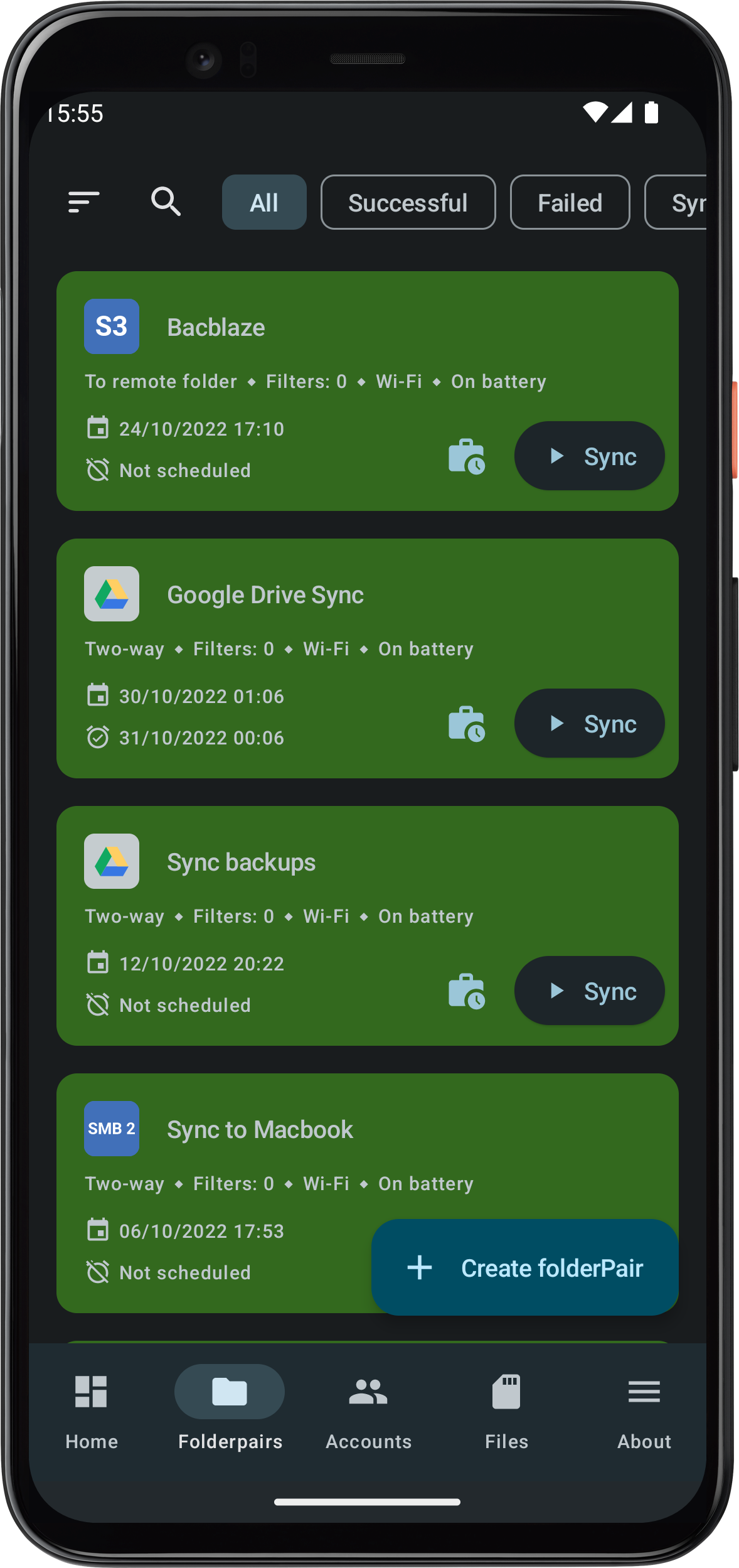The image displays a smartphone interface with a sleek design featuring rounded corners and a distinct top glass screen. The top-left corner shows a full Wi-Fi signal, while the top-right corner displays a fully charged battery icon. Beneath these, the layout includes three distinct sections. 

First, there's a magnifying glass icon followed by a gray square labeled "All" on the left side. Adjacent is a rectangle displaying the text "Successful" and "Fail" beneath it. Below, a green square labeled "S3" is visible alongside details like "Backlight," "Terminal folder," and "Filter is 0." 

Further indicators include "Wi-Fi on battery: 24/10/1 22 70 10" and a note stating "Not scheduled." Another green square labeled "Google Drive sync, 2-way" shows similar details: "Filter is 0, Wi-Fi on battery: 30/10/1 22 1 6 31/10/1 22 0." Another section follows with a green square labeled "SMB2," indicating "Sync to MacBook, 2-way" with "Filter is 0, Wi-Fi on battery: 26/10/1 22 17 53, Not scheduled."

At the bottom of the screen, a blue rectangle features a plus sign along with a gray folder icon denoted "Pair." Surrounding options include "Home, Folder pairs, Accounts, Files, About." The entire interface overlays a gray background, with a white line at the very bottom and a camera icon positioned at the very top.